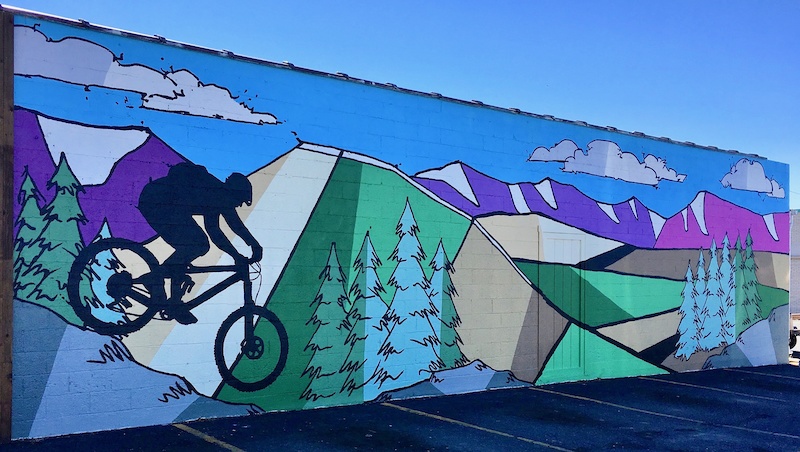The image features a vibrant mural painted on the side of a brick building adjacent to a parking lot, with clearly marked parking lines in front of the wall. The mural depicts a colorful outdoor mountain scene under a blue sky scattered with clouds. The mountains, displayed in a range of hues including purple, pink, green, and brown, utilize block coloring techniques. Among the mountains, numerous green pine trees or spruces are scattered, enhancing the natural motif. In the lower left corner, there's a silhouette of a man riding a mountain bike downhill, complete with a helmet and a backpack. This shadowy figure stands out against the vivid background. The scene is illuminated by sunlight, which casts shadows that suggest it is late in the evening. The entire artwork adds a captivating and scenic element to the small building’s exterior.